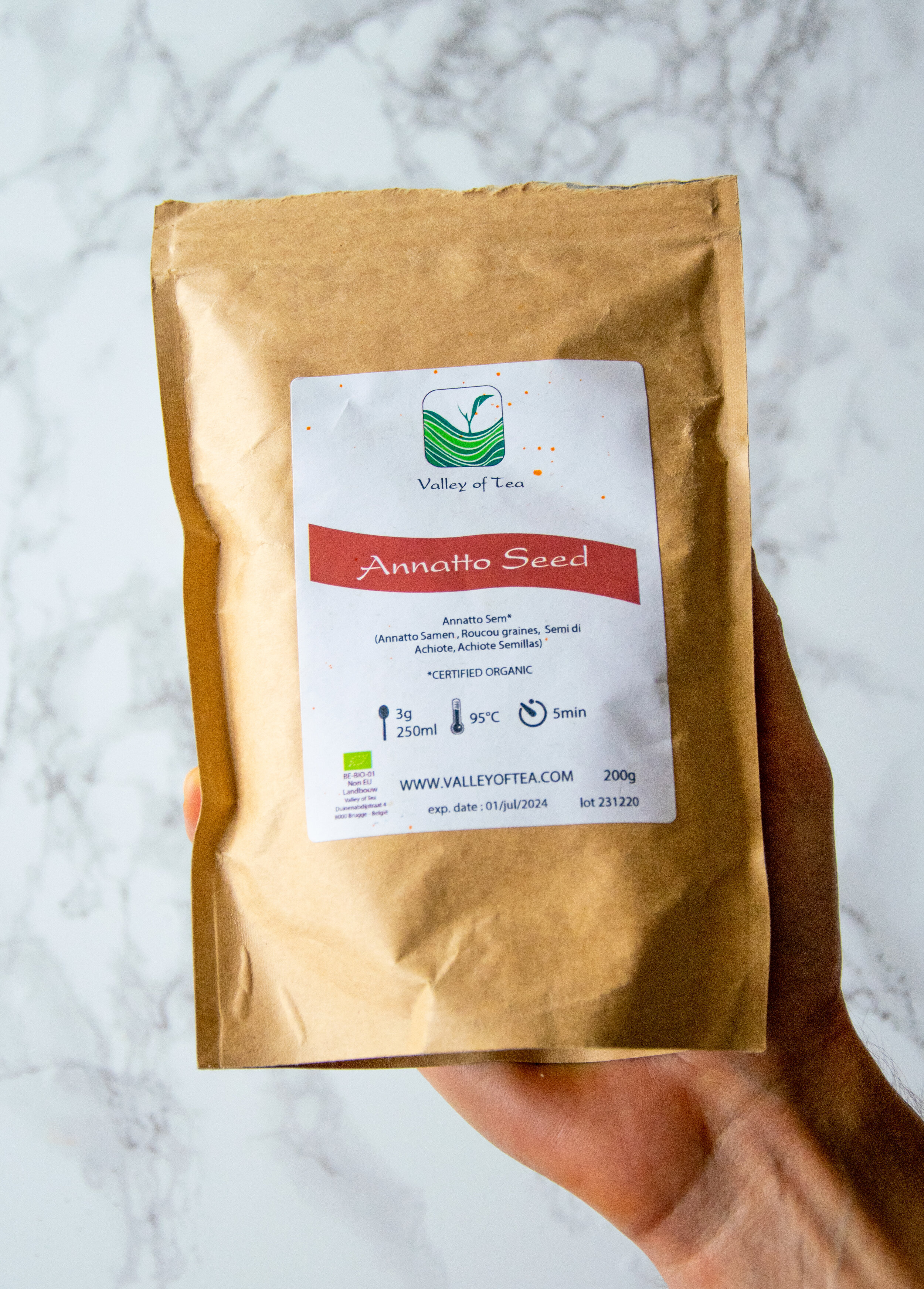In this photograph, a hand with fair skin holds a manila yellow tea bag labelled "Valley of Tea." The hand appears palm up, with the bag positioned in front of a white and gray marble background. The bag, resembling a manila envelope with a seal at the top, features a white sticker on the front. This sticker displays a green logo resembling a flowing valley with a tea leaf, and contains the text "Valley of Tea" in a striking font. Below the logo, a red banner reads "Annatto Seed," indicating the type of tea.

Additional details on the sticker include certification of the product as organic, preparation instructions suggesting 3 grams of tea per 250 milliliters of water heated to 95 degrees Celsius for 5 minutes, and the website www.valleyoftea.com. The package weighs 200 grams, with the expiration date listed as July 1st, 2024, and the lot number as 231220. The label features bold black text and includes informative icons for brewing guidance.